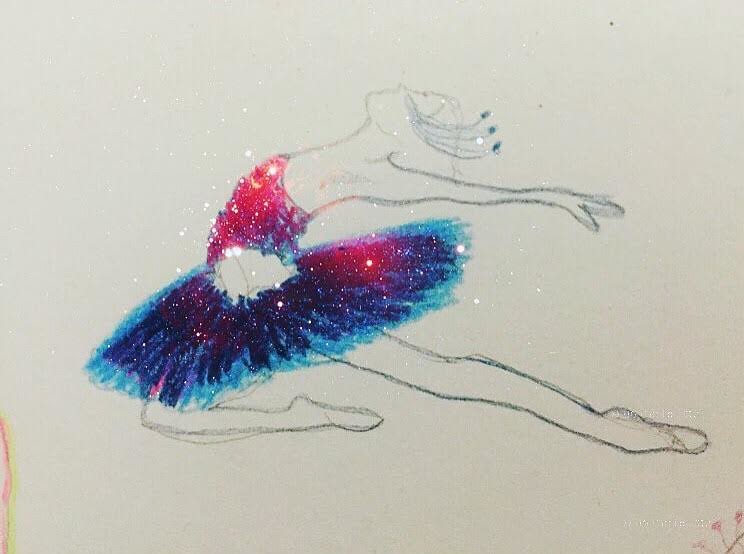This is a detailed drawing of a ballerina captured in mid-leap, rendered in pen on white paper. The ballerina is depicted with a combination of striking colors and intricate details. She wears a tutu that transitions from deep turquoise and purple to a vibrant red at the top, adorned with sparkling white dots that resemble twinkling stars. Her top is a more intense red, shimmering with the same sparkly pattern.

Her pose conveys dynamic movement; she has one leg extended straight behind her, illustrating a realistic ballet shoe, while the other leg is bent at the knee with toes pointed backward. Her body is arched backward with an arm extended gracefully behind her, fingers outlined in fine detail. Her head is tilted upward, revealing grayish outlines of her face, neck, and chest, contrasted with a darker pencil shading on her extended arm and back leg.

The ballerina's hair features three long bluish braids that cascade down and extend to the right. She dons a silver and blue crown that adds a regal touch to her ethereal appearance. The tutu’s dark blue core lightens to a sky-blue trim, further embellished with sparkling white dots, giving it a galaxy-like aesthetic. Surrounding the main image, the bottom left corner of the paper has a line in pink or peach with neon bright yellow, while the bottom right corner features thin lines ending in red circles.

Overall, the drawing is a captivating blend of sharp realism and imaginative color, capturing the elegance and grace of the ballerina in a moment of suspended flight.